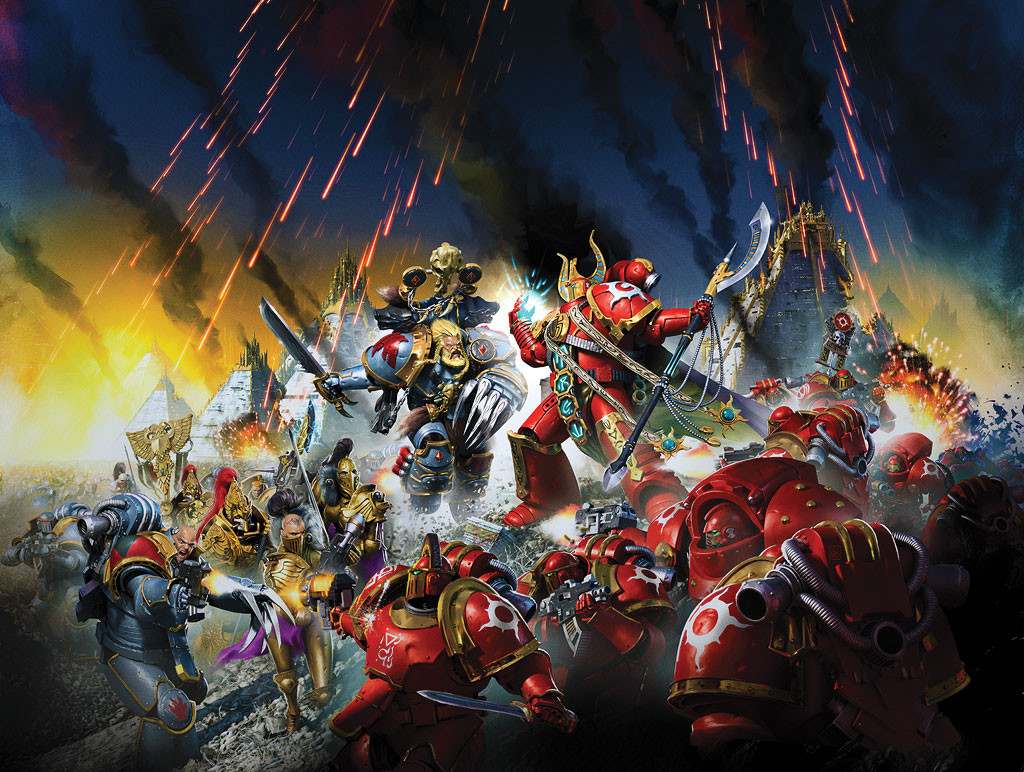The image portrays a dramatic digital artwork reminiscent of an oil painting, capturing an intense battle among numerous superheroes. Central to the composition is a triangular formation of superheroes clad in red armor, engaging in fierce combat with adversaries. The backdrop features a dark, medium-blue sky punctuated by yellow explosions and streaks of black smoke from weapon fire, intensifying the chaotic atmosphere.

Positioned on the right side, a contingent of heroes wearing red armor clashes with opponents in black and gold armor on the left. Dominating the center are two primary figures, highlighted by a blazing white explosion behind them, making them stand out vividly. The figure on the left dons an outfit somewhat resembling Spider-Man’s, complete with a trident motif on the head. Opposite him is a figure in blue armor, adorned with a red emblem on the arm.

Scattered throughout the scene are various other characters in disarray, emphasizing the warlike tumult of the battlefield. The composition effectively conveys the ferocity and disorder of this superhero skirmish, with each side clearly defined by their distinctive armor and positions.